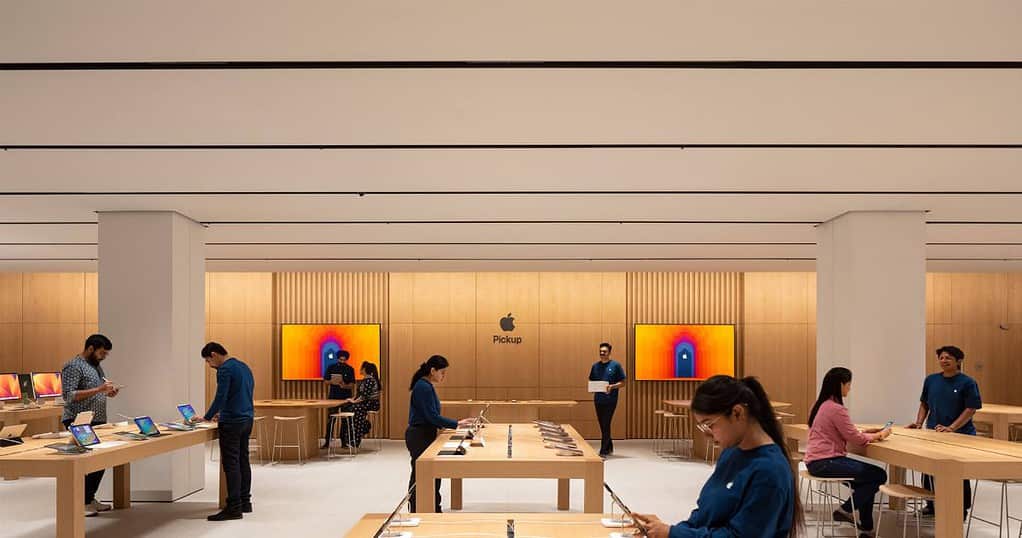The image depicts a bustling retail store, characterized by a modern, open layout. The store features an Apple pickup area flanked by two flat-screen TVs mounted on the walls. The space extends into what appears to be a hallway on either side, with two metallic poles punctuating the scene. The flooring is a pristine white, while the ceiling displays a subtle beige hue, mirrored by the color of the poles.

In the foreground, a woman is seated in a chair, engaged in conversation with a salesman who is attentively holding an iPad. Nearby, another salesman, also with an iPad in hand, is walking towards a woman examining cell phones, possibly to assist her. The area is lively with activity; another woman is intently browsing cell phones, while a man inspects an iPad with the aid of another salesman. Close to them, a third man stands nearby, suggesting he's next in line for service.

Further into the store, a woman is comfortably seated in a chair and a man is situated at a table, engrossed in his task while another man stands adjacent to him, likely providing assistance. The overall scene captures the dynamic interaction between customers and sales staff within the sleek, organized environment of the store.